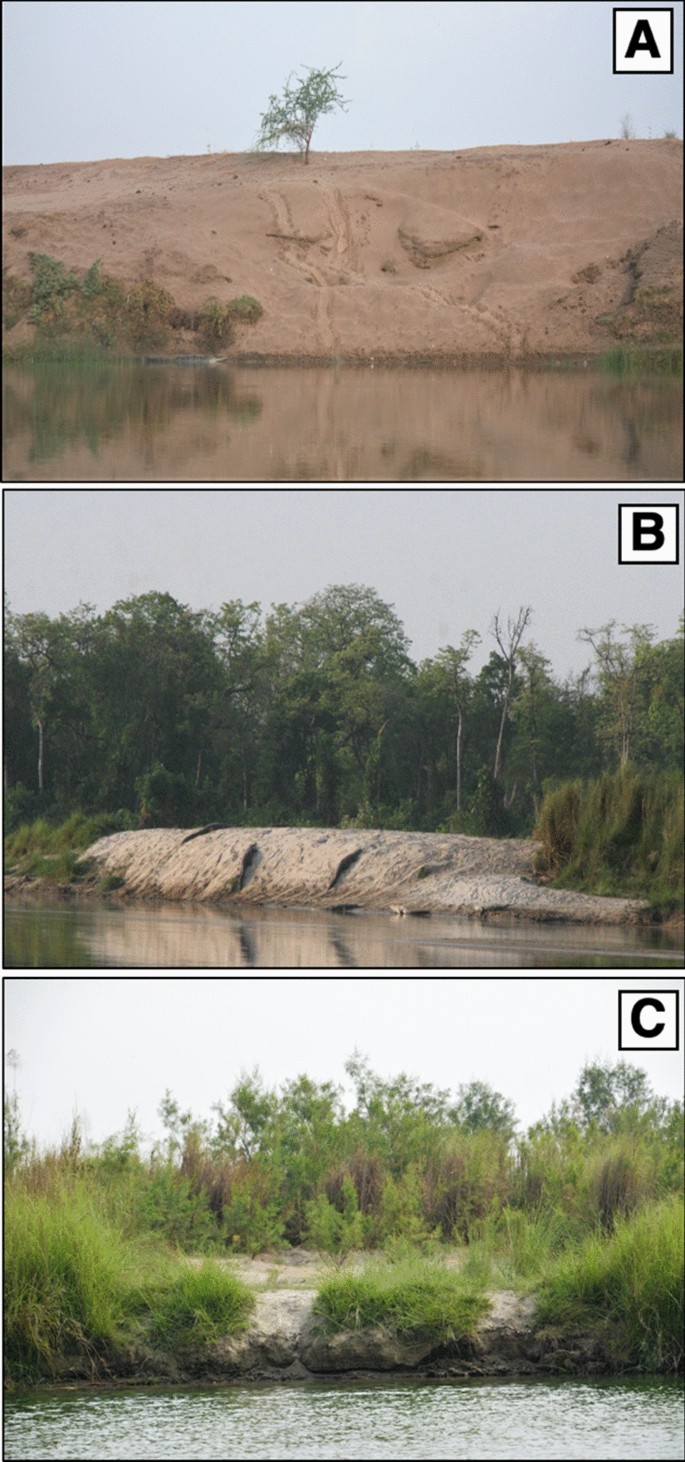The image is a panel of three vertically aligned photographs, labeled A, B, and C in bold black text set within small white squares located in the upper right corner of each photo. Each photograph depicts distinct shoreline landscapes characterized by different compositions of water, slopes, and vegetation.

The top photograph (labeled A) features a body of water leading to a sandy slope dotted with sparse bushes and a single tree. Behind this slope, the terrain rises gently, showcasing the beginning of a larger landmass.

The middle photograph (labeled B) captures another body of water, this time contrasted by a steeper slope that hosts lush, larger green trees. This slope appears less sandy and more vegetative, providing a stark contrast to the simpler landscape above it.

The bottom photograph (labeled C) displays a body of water adjacent to a significantly eroded and flat sandy area. This shoreline is adorned with green shrubs and miscellaneous foliage, indicating a mix of natural erosion and vegetation growth.

Overall, the panel emphasizes the varying types of shorelines and their respective vegetations, with consistent elements of water, slopes, and greenery.